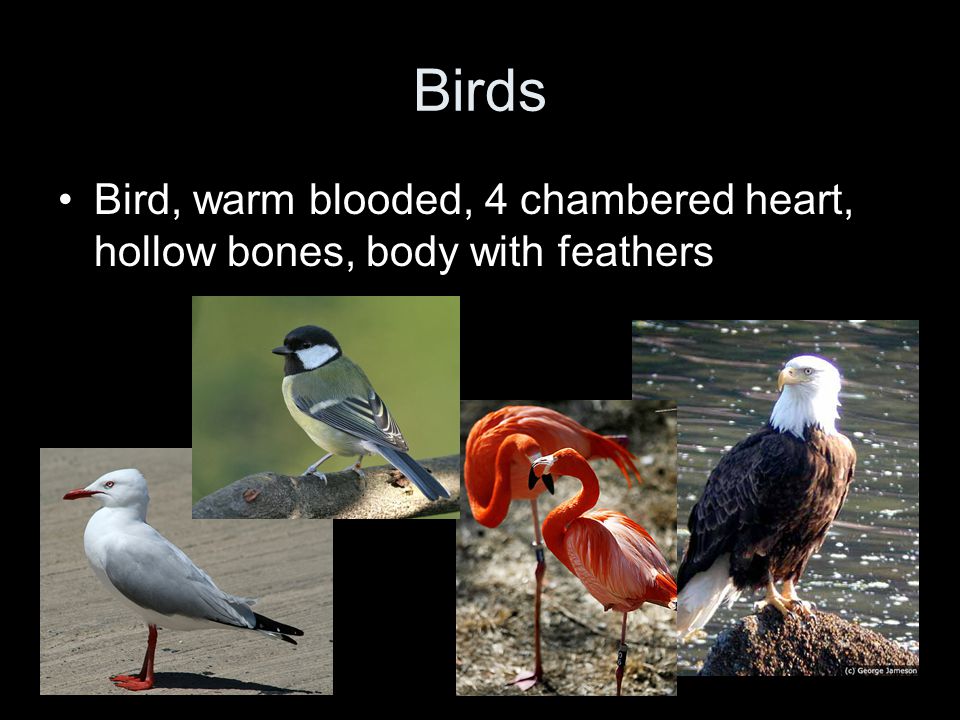The image is a composition on a plain black background featuring the word "birds" prominently at the top in white text. Beneath this title, there is descriptive text also in white, listing characteristics of birds: "bird, warm-blooded, four-chambered heart, hollow bones, body with feathers." The main section of the image consists of four distinct bird photographs, aligned horizontally beneath the text. 

Starting from the left, the first photograph depicts a white bird, likely a seagull, exhibiting shades of gray and black with red-orange feet and beak. The second photograph shows a small bird with a black and white head, yellow belly, and a bluish-greenish-brown back, probably a finch, perched on a branch. Next, the third photograph features two flamingos, characterized by their signature pink color, standing on one leg. The final photograph on the right displays a majestic bald eagle with its distinctive white head, yellow beak, brown body, and white tail, perched on a rock near water. The overall setting for the birds is outdoors, capturing elements of their natural habitats.